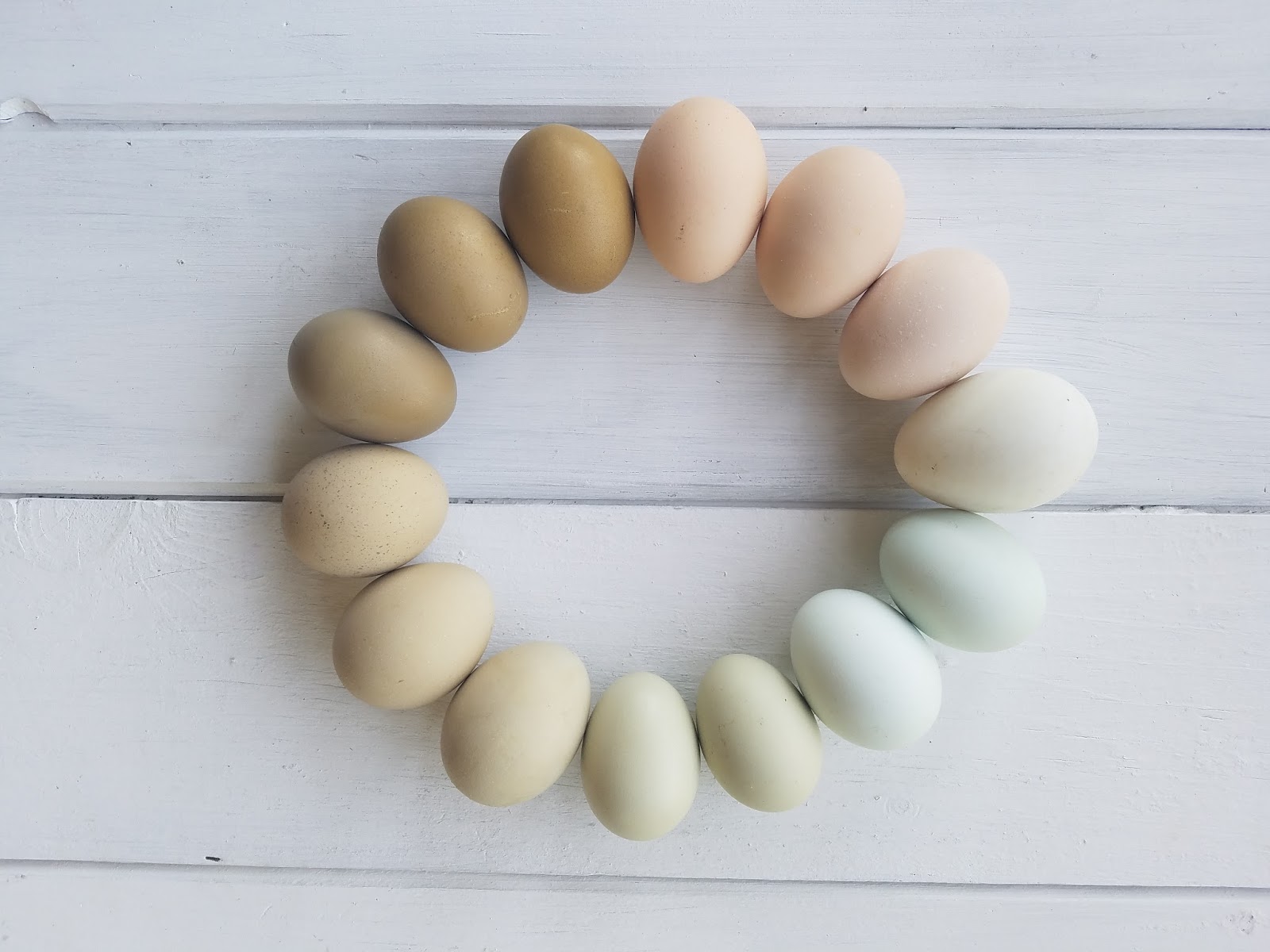The photograph showcases 14 eggs meticulously arranged in a circular formation on a wooden surface that has been painted white. The eggs, varying slightly in size, are each pointed inward with their narrower ends, contributing to a visually engaging composition. 

This ring of eggs exhibits a gradient of colors, forming a subtle yet distinct spectrum. Starting from a peachy-colored egg at the top, the eggs transition clockwise through lighter shades until becoming almost white. Following this, the hues shift to a pale bluish tone, then progress through various shades of brown, until finally returning to the initial brownish hue. Notably, the bottom of the circle features a subtle mint green egg, adding to the diversity of colors.

The wooden surface beneath the eggs, resembling a weathered picnic table or siding, features irregularities where the white paint appears worn thin in places, further enhancing the rustic charm of the image. This detailed and colorful arrangement of eggs offers a captivating display of natural variation and beauty.